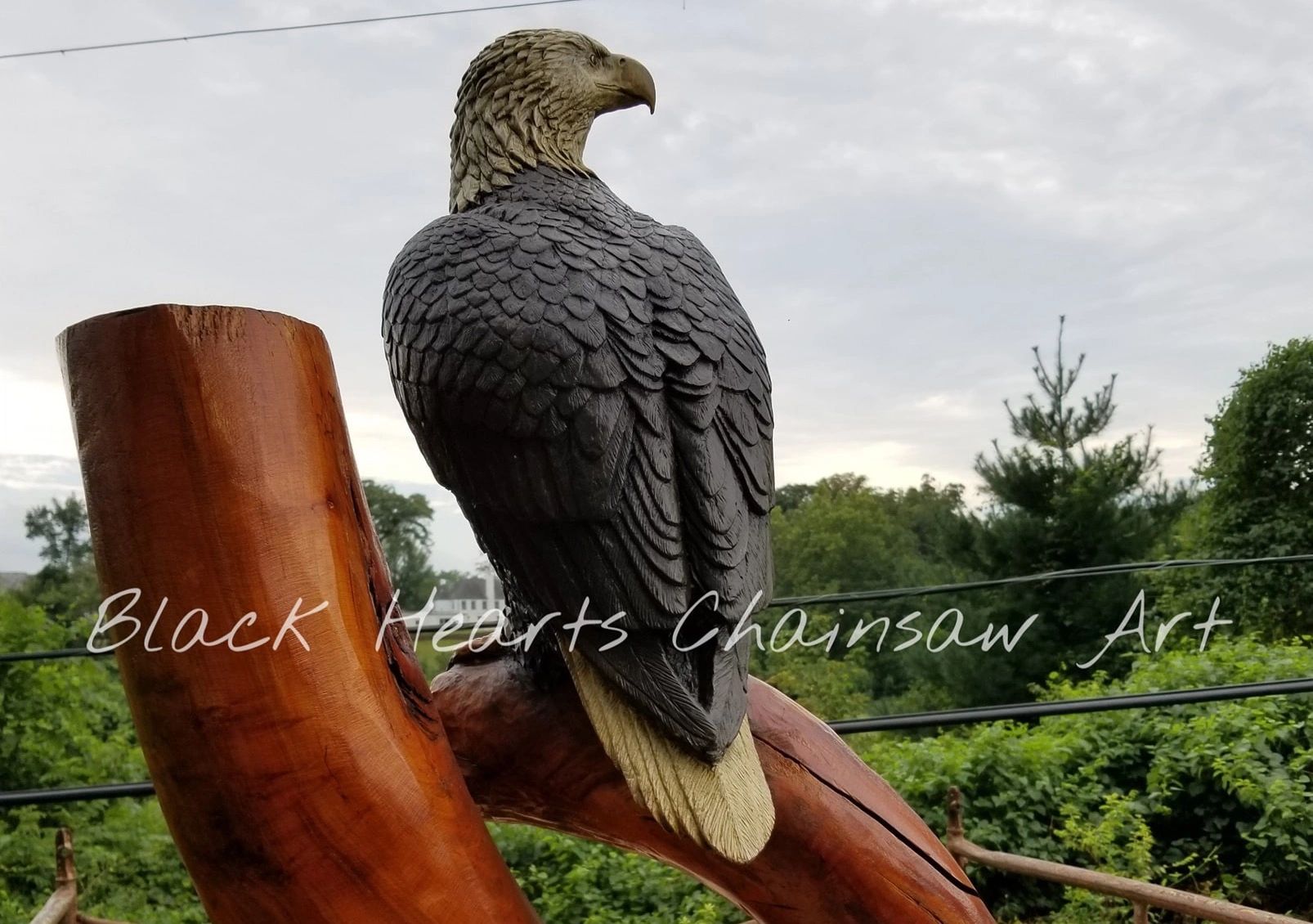The image is a horizontal, rectangular outdoor photo prominently featuring a detailed eagle sculpture. The sculpture, likely carved from wood, showcases a predominantly black body with white accents and intricate feather details, suggesting it may be a chainsaw art piece. The eagle is perched on a similarly carved branch, and it gazes off to the right side of the image. The background is filled with green tree tops and the faint presence of power lines, all set against a cloudy, overcast sky of white or light gray hues. Across the photo, in white letters, is the text "Black Hearts Chainsaw Art," indicating the nature of the artwork.